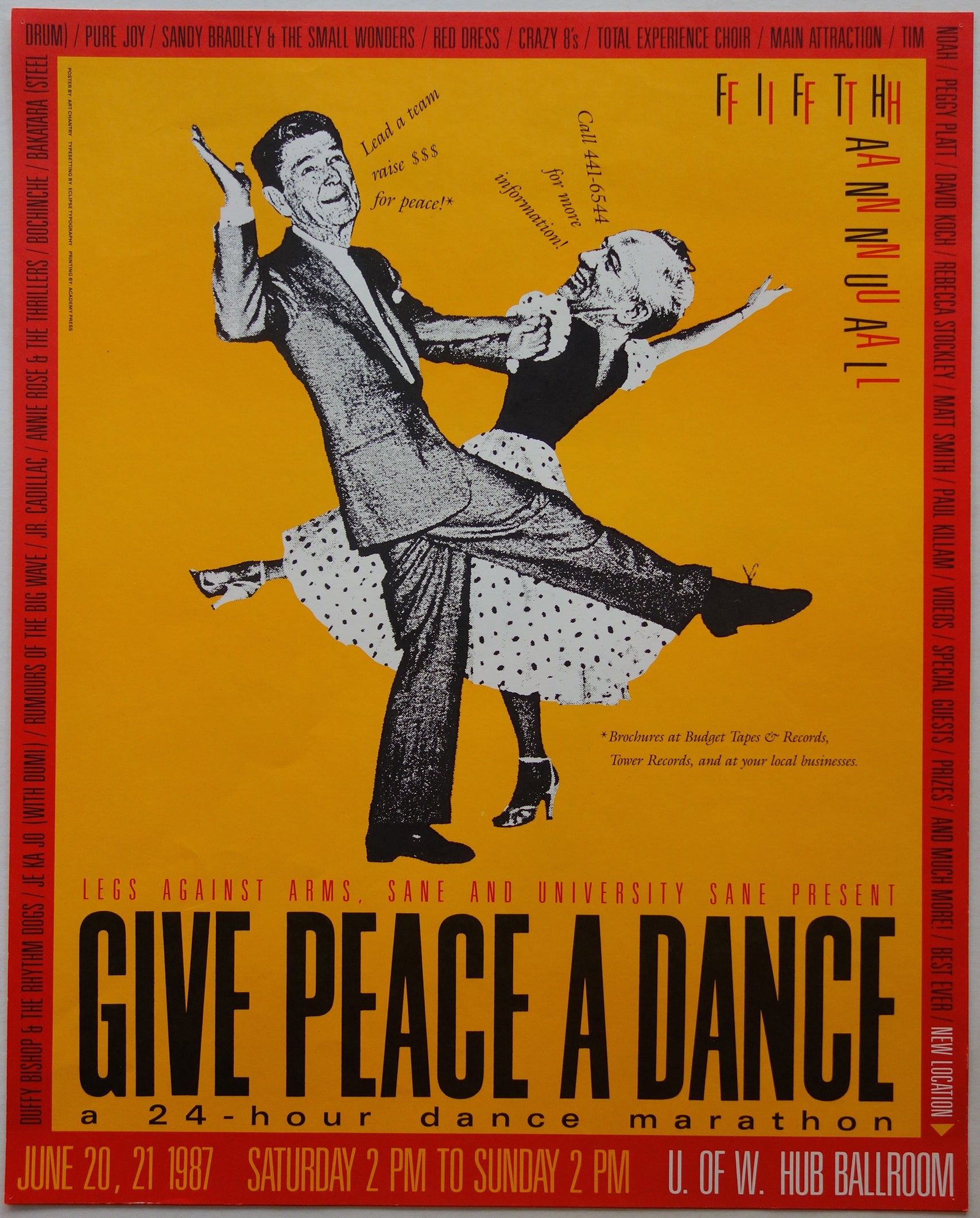This vibrant flyer is an advertisement for a "Give Peace a Dance" 24-hour dance marathon event held at the University of Washington HUB Ballroom. Dominated by a yellow background and enclosed by a red border with black text, the poster is visually striking but challenging to read due to the black text on a red border. 

At the top, red text states "Legs Against Arms" and mentions an unclear reference to "sane and university sane present." Below this heading is a quirky black-and-white photomontage featuring Ronald Reagan dancing with Mikhail Gorbachev, as their heads are superimposed onto the bodies of a man in a suit and a woman in a 1950s-style polka-dot dress. Reagan's head is looking upwards with his right arm at a 90-degree angle, while the Gorbachev figure is extended towards the top right corner.

Sprouting from Reagan's mouth are the words "Lead a team, raise $$$ for peace," while the Gorbachev figure’s speech bubble reads "Call 441-6544 for more information." Additional event details, like a list of performing bands ("Pure Joy, Sandy Brady, Small Wonder, Red Dress, Crazy 8, Total Experience Choir, Main Attraction, Tim's Noah") run along the border.

At the bottom in large black letters, the poster declares "Give Peace a Dance," followed by "A 24-hour dance marathon." Further down, it notes that the event will occur from Saturday, June 20th, 1987, at 2 p.m. to Sunday, June 21st, 1987, at 2 p.m., marking the fifth annual occurrence of this dance marathon. The U of W HUB Ballroom is mentioned in white text against the red banner near the bottom. Lastly, there is an asterisk noting that brochures are available at local businesses and record stores.

Through its eclectic mix of playful imagery and retro flair, this poster whimsically promotes a significant dance event, aiming to unite participants in a frenzy of fun and fundraising for peace.